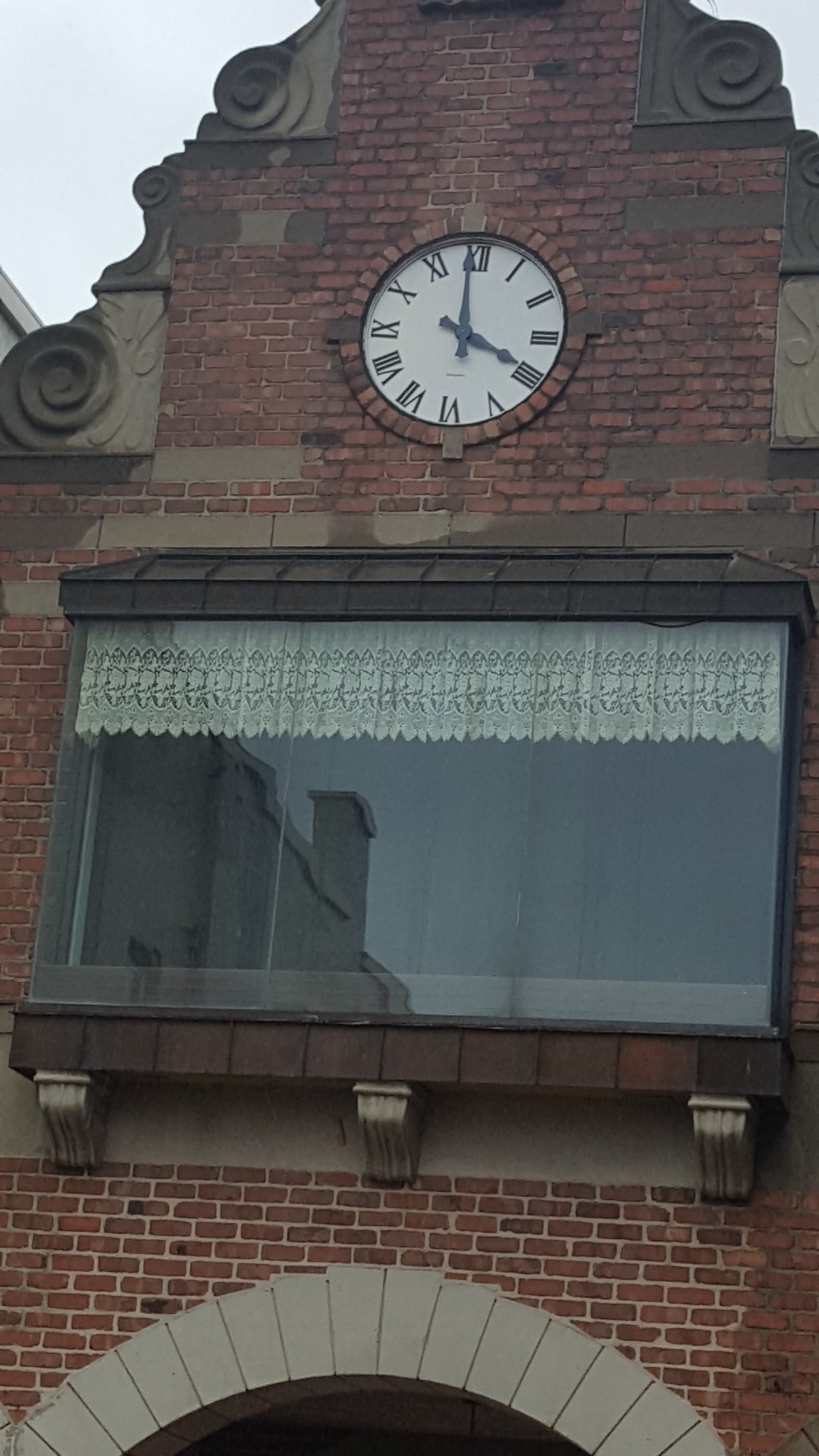This photograph captures the upper section of a classic red brick building, likely part of a historical structure. The lower portion of the image showcases a gray stone archway with detailed masonry. Above this archway, a large window is prominently featured, adorned with an intricate, frilly design along the inner top border. Ascending further, the photo reveals more of the red brick masonry leading up to the roofline. The roof itself has decorative swirl-like architectural elements, adding an elegant touch. Centrally situated above the window is a round, white clock. The clock face displays black Roman numerals and matching black clock hands, standing out strikingly against the weathered brick backdrop. The glimpse of the sky above suggests an overcast, rainy day, contributing to the atmospheric feel of the scene. This image likely captures the upper façade of a clock tower or similar historic building.